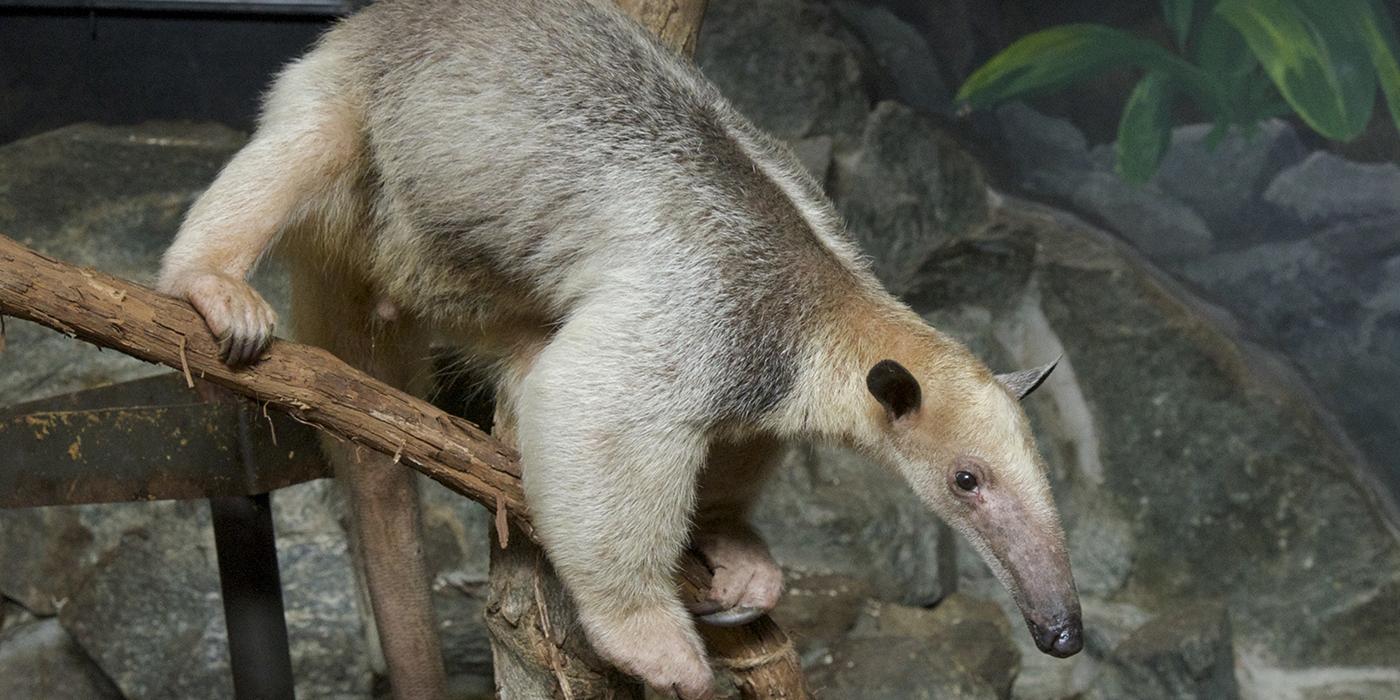The image captures a detailed scene featuring an anteater, identifiable by its long snout and pointed ear, as it stands on a wooden railing. The anteater sports a striking gray coat that transitions into a black color at its extremities. The animal is positioned such that its right foot is on top of the railing while its left foot remains at the bottom, giving the impression that it might be leaning or exploring. The creature appears to be gazing downwards, potentially looking for food. The surrounding environment includes large grayish rocks and green plants cascading over them, suggesting a naturalistic setting that could either be a wildlife reserve or a zoo.